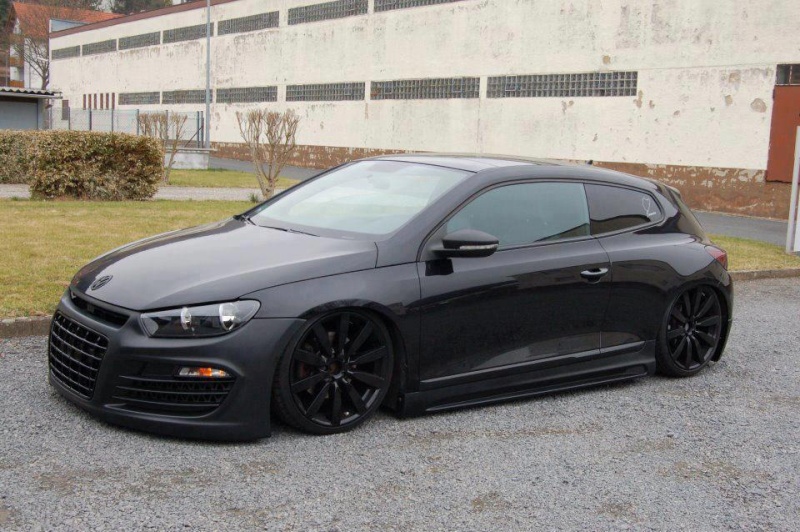An all-black, modified hatchback is parked on a gray tar road in front of a large white building. The vehicle features black spoke rims and black wheels, giving it a sleek, low stance that nearly touches the ground. The front headlights are tinted with a black hue, blending seamlessly with the car’s classy black paint job. The driver's side window remains clear, while the smaller rear side window is tinted black. A distinctive white line marks the driver's side mirror. In the background, a mix of dry yellowish grass and green patches is bordered by a bush and two dead trees. The large building, resembling a cement factory, stretches across the backdrop with its white walls, small horizontal windows arranged in two rows, and features white partitions between the panes. To the top left, the corner of a reddish-brick building is visible, adding contrast to the scene.